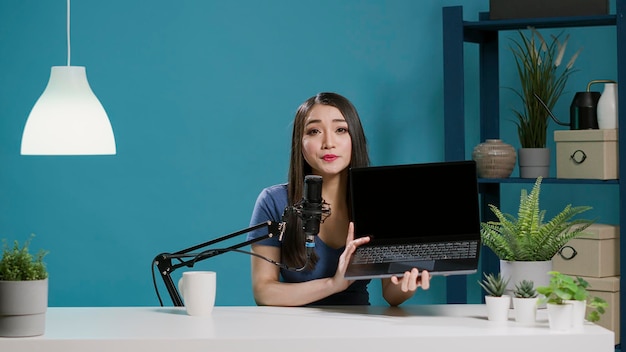In the image, a young Asian woman with long, straight black hair and red lipstick is seated behind a white desk. She is holding up a black laptop with a black screen and grey keypad, presenting it to the camera as if demonstrating or explaining something. The woman, dressed in a blue top, is actively engaging with the camera, which is mounted on a black stand and equipped with a fuzzy black microphone.

The setting appears to be an office or home workspace characterized by various thoughtful details. To her left, a white pendant light with a glass shield hangs from the ceiling. Surrounding her on the desk are several potted plants, including green ferns in white pots and a dark green cactus in a grey pot, adding a touch of greenery to the scene. A white ceramic mug rests on the desk beside her.

Behind the woman, the wall is a vibrant blue, creating a striking backdrop. Positioned on a shelf to her right are an assortment of items: a potted plant with fine green leaves in a grey pot, a vase, a beige box, a black air freshener, a white ceramic bottle, and several jars and additional brown boxes. This well-organized shelf adds depth and context to the setting, evoking a professional yet homey atmosphere.

Overall, the image captures a highly detailed and vibrant scene, presenting the woman in an engaging and professional light.